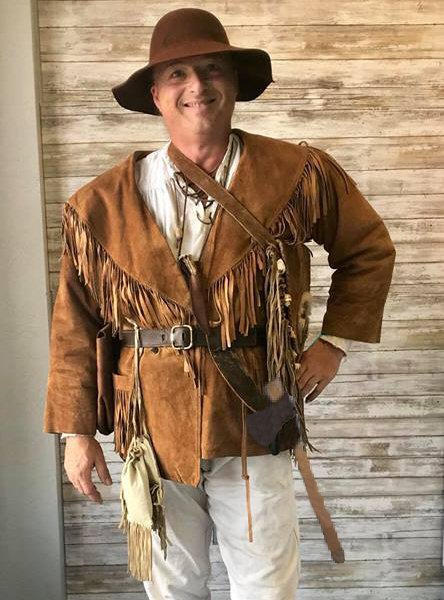This vertically oriented, full-color photograph captures a cheerful man dressed in an elaborate period costume, evoking the style of a Davy Crockett explorer. He stands in front of a distressed wooden slat wall that features light brown, dark brown, and lighter brown streaks, with a small section of a plain white wall visible on the left. The man's head reaches the top of the photograph, and the image extends down to slightly below his knees.

The man, who has white skin, wears a wide-brimmed, floppy dark brown leather hat. His light brown suede jacket features a large shawl collar adorned with long fringe, which also decorates the pockets. Underneath the jacket, he sports a white shirt with brown laces that tie at the neck. His waist is cinched by a brown leather belt from which a cream-colored, fringed pouch hangs on his left side. On his right side, a strap hides partly under his jacket and holds a small bag under his arm. He also has an axe secured in his belt. Completing his outfit, he wears cream-colored pants. The man poses with his left hand resting confidently on his hip, smiling directly at the camera. The overall scene is a stylized representation within a setting aimed at photographic realism.